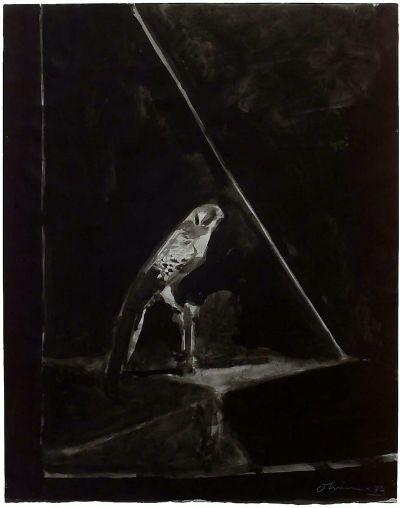This detailed and moody artwork, likely created with black ink or charcoal, presents a striking monochromatic scene. Dominated by a somber black background, the painting features a bird with a rounded head and small, curved beak resembling a falcon, perched on a flat, dark gray surface. The bird, predominantly light gray with dark speckles on its wings and a long, dark tail, contrasts sharply with its environment. The composition is further dramatized by a white diagonal line that stretches from the top left to the bottom right of the image, accentuating the bird's somber isolation. The artist's signature, rendered in white cursive at the bottom right, remains illegible. The overall atmosphere is dark and foreboding, with minimal light penetrating the scene, evoking a sense of loneliness and confinement for the bird amidst the shadowy expanse.